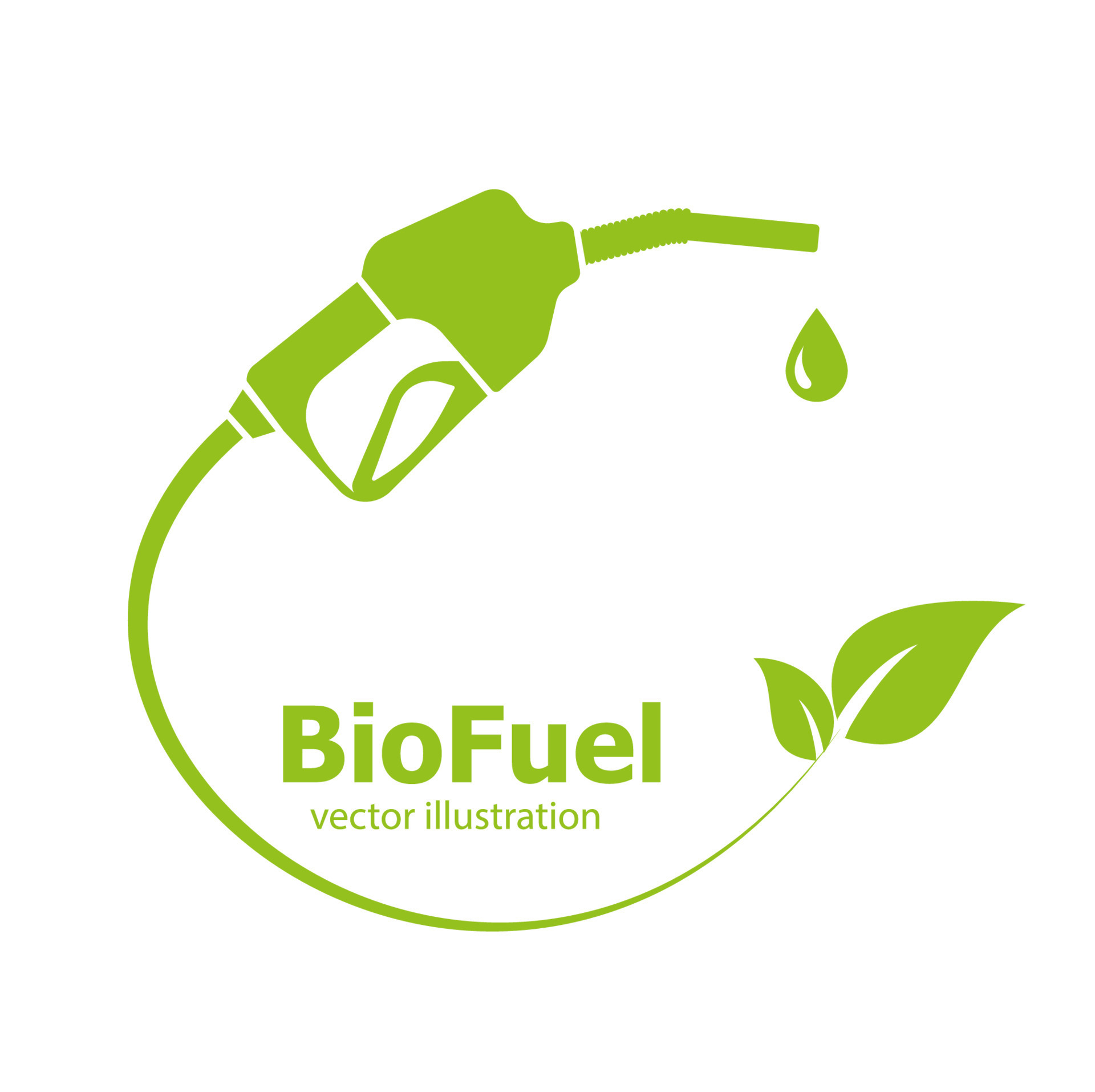This image is a green-themed clip art icon or logo of a gas pump on a white background. The hose of the gas pump curves initially to the left and then back around to the right, transforming into the stem of a plant with two leaves at the end. A single teardrop-shaped droplet is depicted dripping from the pump. In the center of the image, the text "biofuel vector illustration" is written in matching green, indicating its eco-friendly focus and potential use as a biofuel symbol. The overall design is intended as a stock image or example for use by graphic designers and not an existing brand.